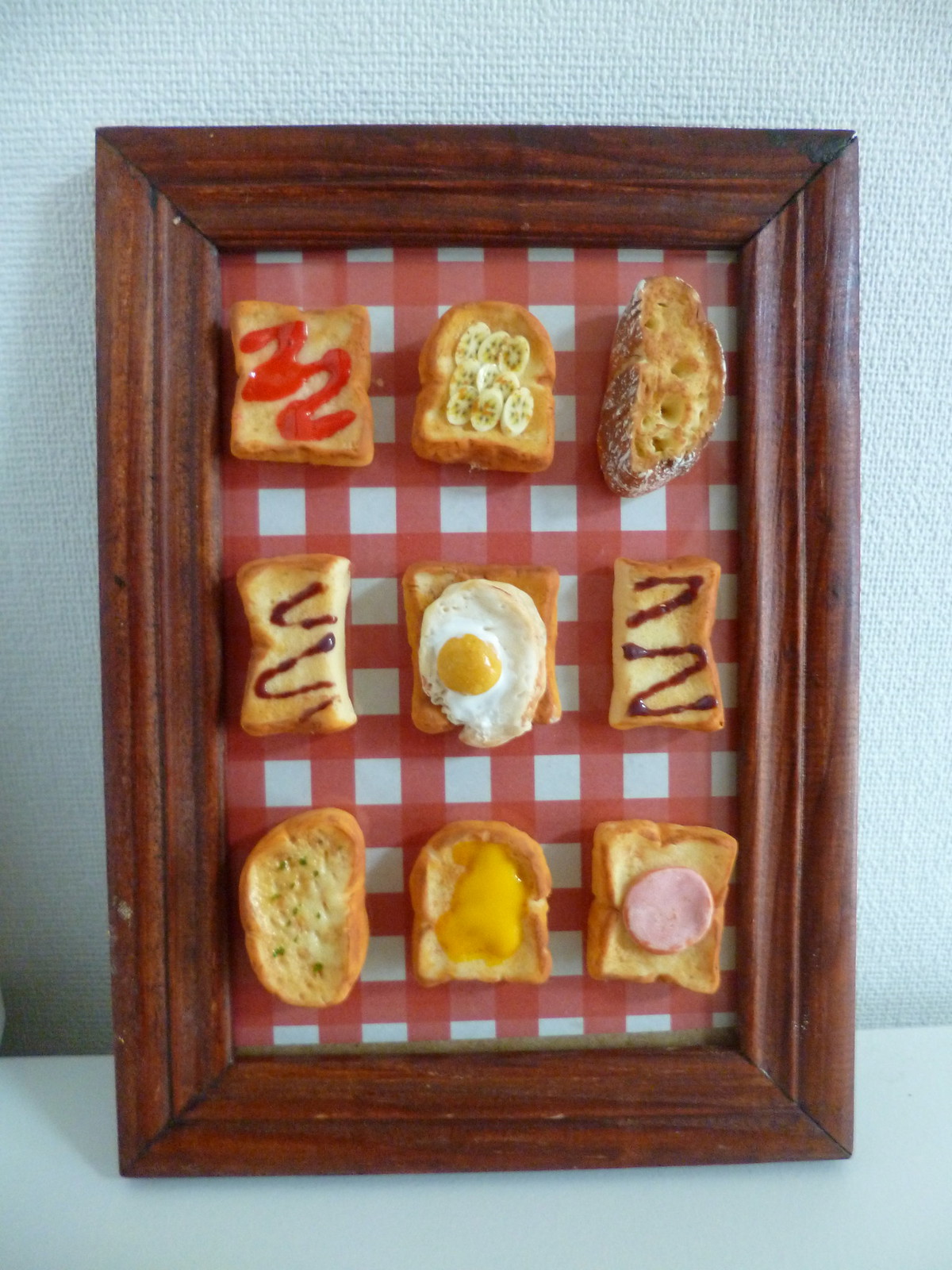This image showcases a meticulously framed display of polymer clay breakfast toast items, arranged in a 3x3 grid. The frame is made of elegant cherry wood, and the backdrop is a red and white gingham pattern, reminiscent of a classic checkered tablecloth. The entire piece is set against a plain white background, potentially with a subtle bluish tint.

In the top row, the leftmost piece is a slice of toast adorned with a red drizzle, possibly strawberry preserves or ketchup. Directly to its right is a piece of toast topped with banana slices. The third piece in this row is a crusty slice of bread, likely French or Italian, dusted with white powdered sugar.

The middle row features a piece of toast in the center, topped with a sunny side up egg, showcasing its vibrant yolk. On either side of this toast are halves of a piece of French toast, each decorated with a zigzag of dark red drizzle, possibly grape jelly or jam.

In the bottom row, the leftmost item is a slice of garlic bread, detailed with green seasoning. The middle piece appears to be toast with a yellowish-orange puddle, likely cheese or egg yolk. The final piece in the bottom right corner is a slice of French toast topped with a slice of ham or Canadian bacon.

This arrangement, with its detailed miniature food items, offers a charming and whimsical take on classic breakfast fare, beautifully framed and presented on a white table.